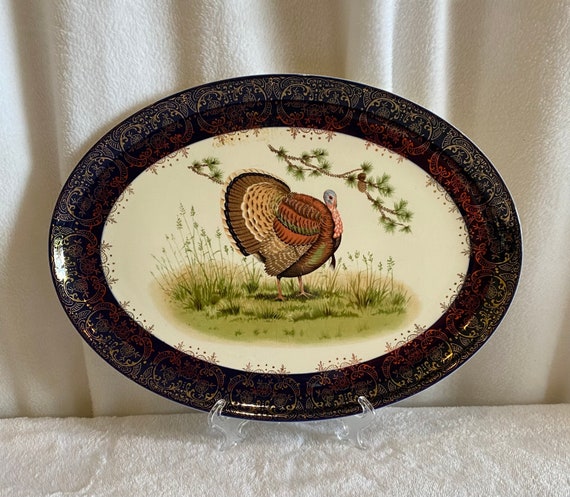This image showcases an ornate, oval decorative plate carefully positioned on a clear glass or plastic stand. The background features both an off-white table cloth and a similarly colored curtain, framing the elegant scene. The plate itself has a striking perimeter, predominantly black with intricate golden embellishments that repeat in a detailed pattern around the edge. The central portion of the plate depicts a vividly painted turkey, characterized by its light brown and red feathers, along with a fan of tail feathers displaying a mix of dark, light brown, green, and white shades. The turkey stands atop a textured green patch of grass, surrounded by small weeds. Overhead, two branches hang down – one smaller and one larger, adorned with either acorns or pinecones. This creates a picturesque, nature-themed scene, masterfully captured on a plate that appears both ancient and artistically rich.